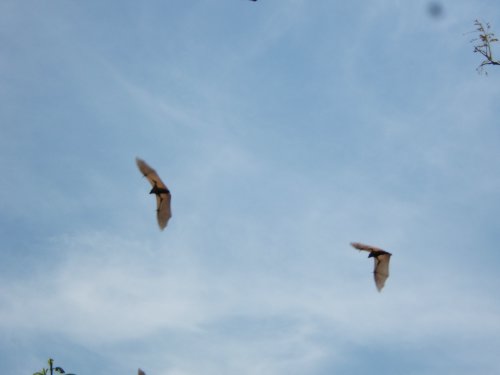This captivating image captures two bats gracefully soaring through a partly cloudy, light blue sky. The bats, identifiable by their translucent wings through which light shines, dominate the scene, moving from right to left. The bat on the left has its wings fully extended, revealing the dark central body and delicate wing structure, while the one on the right has its wings partially closed at a 45-degree angle, as if caught mid-flap. In the background, a small portion of a tree branch is visible in the top right corner, and the faint outline of either the tippy top of another tree or a power line pole can be seen below. The soft, wispy clouds add a serene backdrop to this aerial ballet.